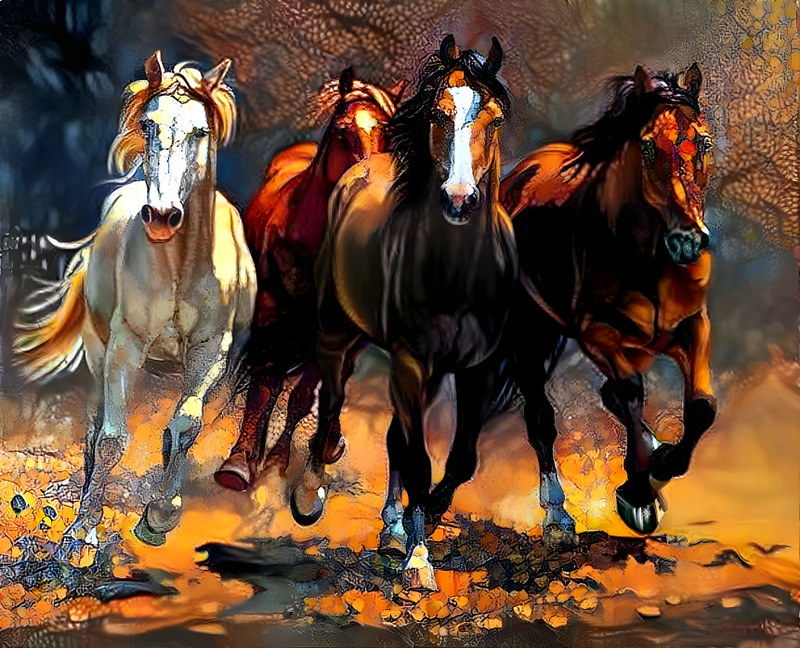This digitally rendered painting depicts four horses galloping towards the viewer, arranged in a two-by-two formation. The prominent horse on the front left has a striking face of white and brown, accentuated by a black mane, while the horse adjacent to it sports a completely brown face and a matching black mane. Behind them, the leftmost horse is predominantly white with a golden-blonde mane, showcasing its lightest hue on its face. The final horse, partially obscured by its compatriots, is a deep chocolate brown with subtle reddish in its coat and black on its legs. The background features vivid strokes of yellow, orange, and hints of tan, suggesting a dynamic landscape possibly resembling sand or earthen tones. The ground beneath them transitions from black and gray to patches of yellow and orange, emphasizing the horses' energetic movement forward.